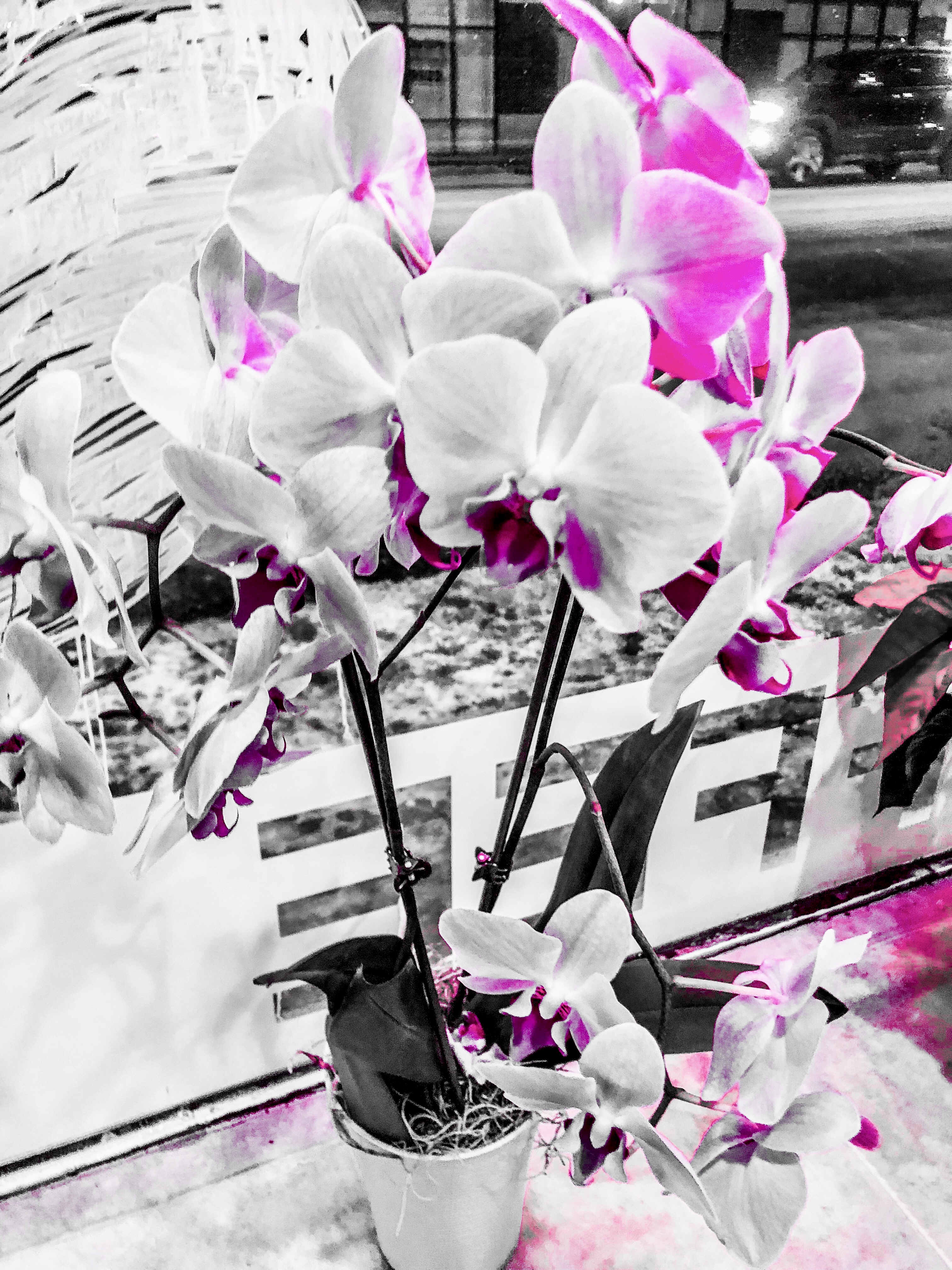The image portrays an outdoor street scene, likely resembling a painting. At the bottom of the image, an asphalt road is visible. In this area, there is a cart filled with flowers, some of which are white with pink and a hint of black, predominantly positioned in the center of the image. The vibrant colors of the flowers contrast against the road. Further details include a cypher-like object on the road, covered in white paint with a splash of pink. In the background, a car with its headlights on is parked, and behind it, storefronts line the street. The top of the image shows various buildings, indicating an urban setting. Although there's no text visible across the entire scene, there's a stencil within the flowers, with indistinct letters such as "E-E-F-F". The overall color palette includes shades of black, white, gray, pink, and purple. The setting appears to feature a wintery mix, with some snow visible on the ground.